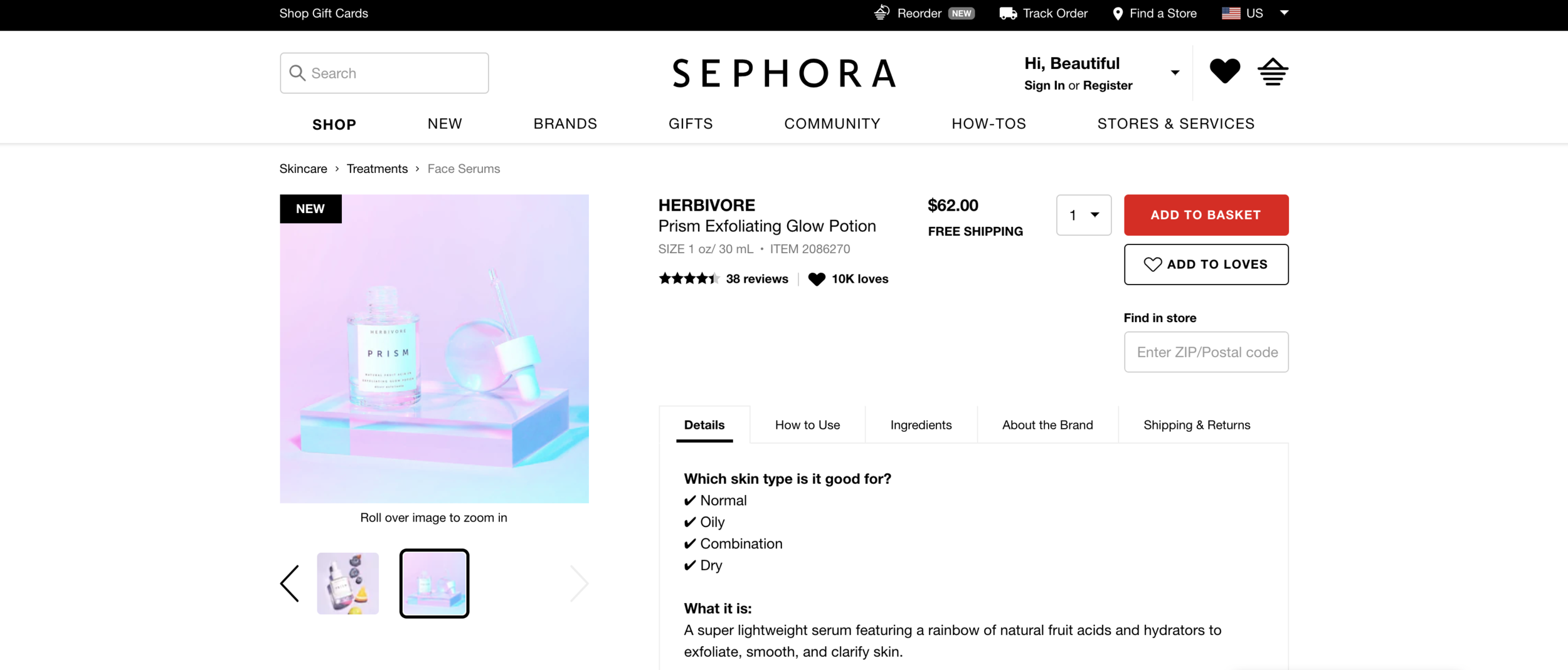This image is a screen capture from the Sephora website, featuring a layout with several key elements. At the very top, there is a black banner. In the upper right corner of this banner, there is a dropdown menu with a US flag, options for "Find a Store" marked by a location icon, "Track Order" with a truck icon, and "Reorder" accompanied by a gray "New" button. On the upper left corner of the black banner, it reads "Shop Gift Cards."

Below this banner, centrally positioned, the logo "Sephora" is displayed in large black font. The left-hand side features a search bar, while the right-hand side displays a greeting "Hi Beautiful" followed by options to "Sign In or Register," accompanied by a heart icon and a basket icon.

Underneath this section are seven main navigation categories: Shop, New, Brands, Gifts, Community, How-To’s, and Stores & Services. 

Centrally below these categories, an item is prominently displayed. The item description reads: "Herbivore Prism Exfoliating Glow Potion - $62 – Free Shipping." There are also interactive options including "Add to Basket," a heart icon for "Add to Loves," and a "Find in Store" feature requiring a zip code. 

On the left side of the product description, an image of the product is showcased, revealing a colorful bottle with a blue and pink color scheme, containing the glow potion.